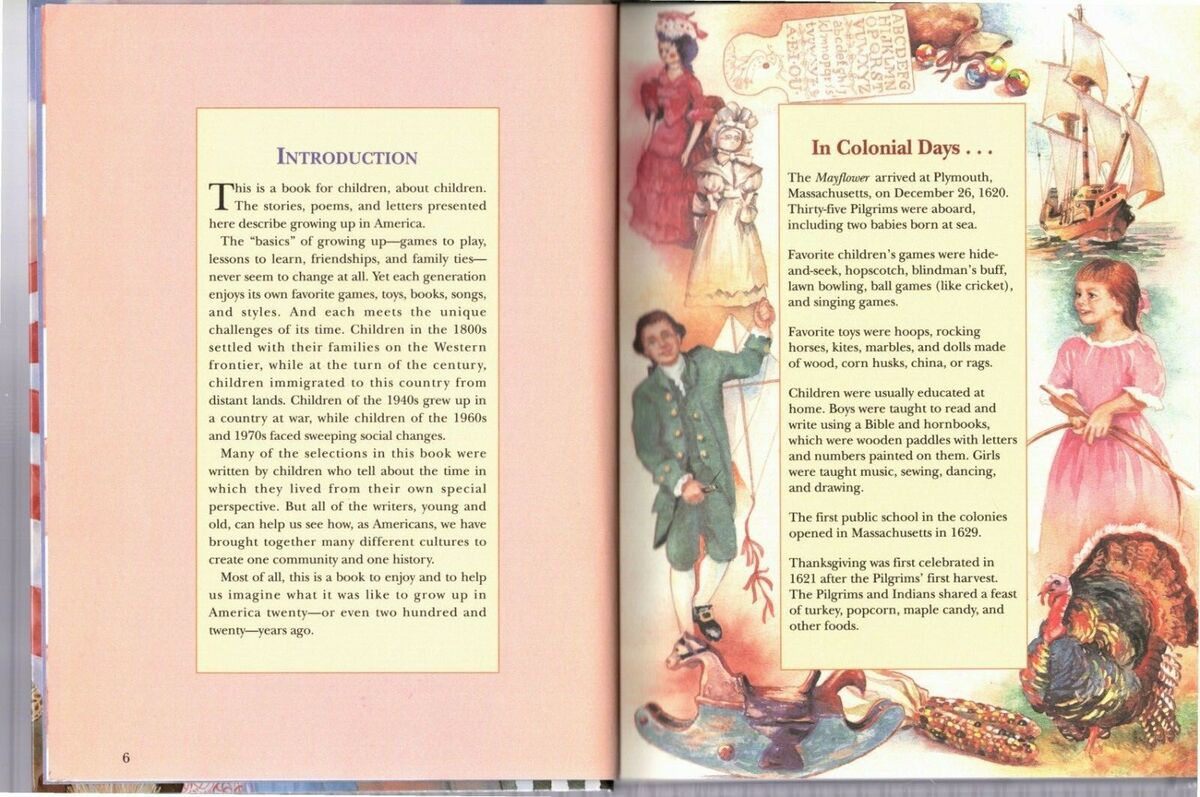The illustrated pages from a children's book depict life in the colonial era for children. On the left, Page 6 features a yellow newspaper clipping style box with the title "Introduction" in purple at the top, followed by black text on a white background. On the right, the page is vividly illustrated. At the top, it starts with the text "In Colonial Days" in a rust-orange hue inside a yellow rectangle, detailing historical facts such as the arrival of the Mayflower in Plymouth, Massachusetts on December 26, 1620, with 35 pilgrims aboard, including two babies born at sea.

The illustration includes various depictions of colonial life: at the center-right, a little girl dressed in a pink colonial dress with ruffled sleeves stands beside a male turkey, symbolizing the Thanksgiving tradition. Next to them lies an ear of multicolored corn. To the left, a wooden blue rocking horse with a small head, a brown tail, and black reins features prominently. Above the horse, an adult male in colonial attire is seen, dressed in a long-tailed jacket with gold buttons, puffy pantaloon pants, and white tights, possibly holding marionette puppets. 

Further up the page, there are white and red-dressed dolls with voluminous skirts and puffy sleeves, resembling colonial dolls, while an alphabet board adorned with different fonts is positioned near the top. A bag of marbles and a few loose marbles sit just below the board. To the far right, an old clipper ship drawn in pencil style, similar to those used by pilgrims, sails the illustrated seas. The art is colorful and detailed, providing a rich visual context for the text on colonial children's lives and activities.